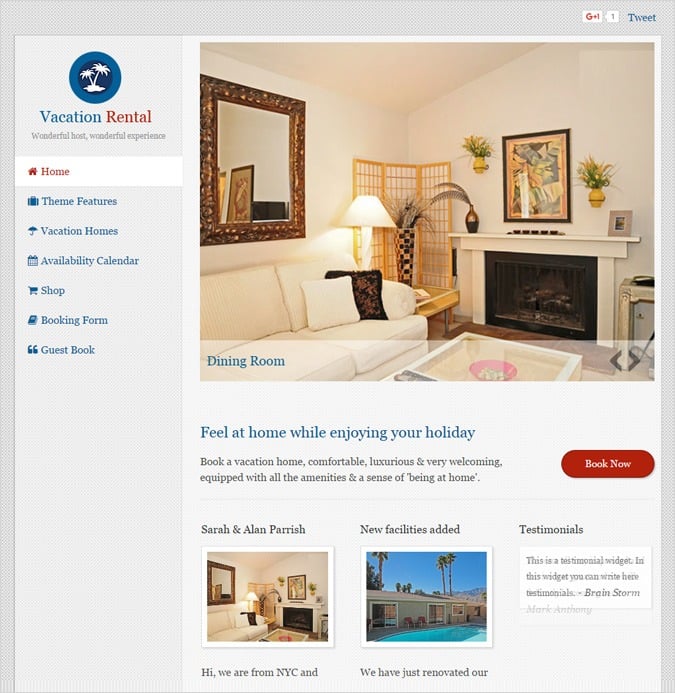The landing page for a vacation rental site features a gray sidebar adorned with a blue logo depicting palm trees at the very top. Below the logo, the words "Vacation Rental" are prominently displayed in blue and brick red lettering. The sidebar menu, predominantly in blue, lists several navigation options: Home, Theme Features, Vacation Homes, Availability Calendar, Shop, Booking Form, and Guest Book, with the selected link highlighted in brick red.

Occupying the main section of the page, there is a large photograph incorrectly labeled "Dining Room," despite clearly showcasing a living room. Beneath this image, a welcoming message reads, "Feel at home while enjoying your holiday," accompanied by a prominent "Book Now" button in red. Further down, additional smaller photos are showcased alongside a link to view testimonials, inviting visitors to explore reviews from previous guests.